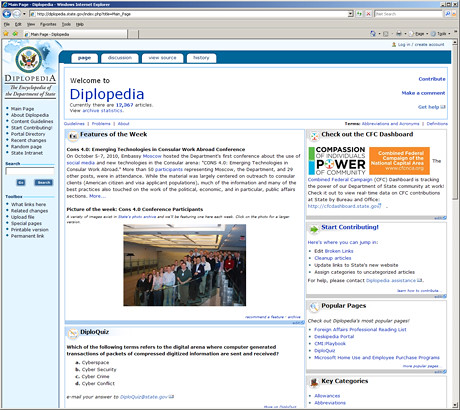The image is a complete screenshot of an early to mid-2000s website displayed on an Internet Explorer browser characterized by its gray background and old-fashioned interface. The headline on the web page reads, "Welcome to Diplopedia," in a blue font, indicative of the period's design aesthetics. Above the headline, the navigational menus have a similarly antiquated appearance, with one tab labeled "History" and the rest illegible due to the small font size. The bottom of the page features a small photograph depicting a large group of people standing in line under a low gray ceiling with what appears to be a large skylight. To the left, the sidebar displays another "Diplopedia" label beneath a circular coat of arms. However, the menu items are too small to discern.